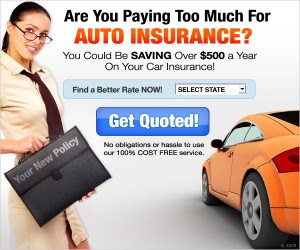In the image, a professional-looking woman stands prominently, holding a sleek black briefcase that has the words "Your New Policy" emblazoned on it. She is donned in a sophisticated tan shirt and skirt, paired with a striking red tie. Her dark hair is neatly pulled back, and she sports glasses that give her a look of serious intent. The woman’s complexion adds to her composed and confident demeanor.

To the right side of the image, an orange car is visible from the back driver's side, showcasing its red brake light and black tires. The vehicle carries a message asking, "Are you paying too much for auto insurance?" It entices viewers with the promise of potential savings—over $500 a year on car insurance—and encourages them to "Find a better rate now."

Beneath this text is a drop-down menu labeled "Select state" with a blue button that has white font saying "Get quoted," inviting users to take action. Below this button, it reassuringly states, "No obligations or hassle to use our 100% cost-free service."

The entire composition is set against a crisp white background, accentuated by a palette of colors including black, red, light blue, dark blue, orange, tan, maroon, and brown. The call-to-action "Find a better rate now" is highlighted in a blue rectangle with rounded corners, tying the elements together in a visually appealing manner.